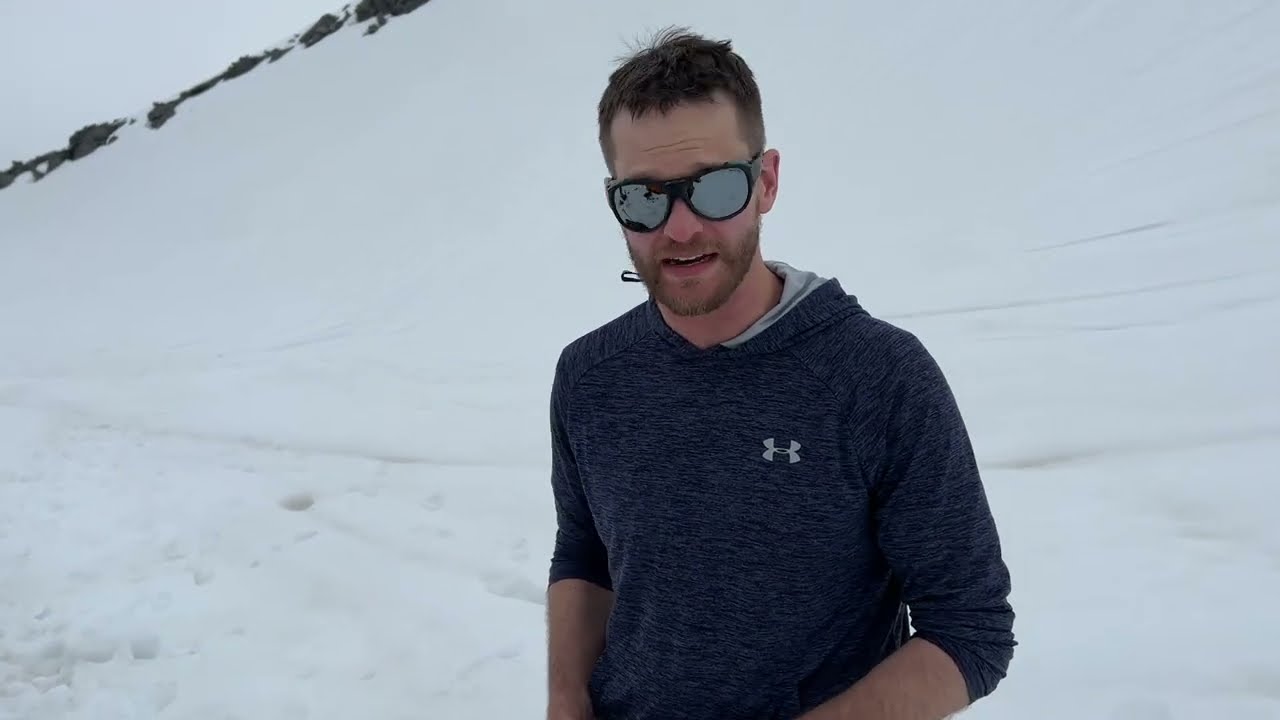In the photograph, a Caucasian man with short dark hair and a beard stands in an extensive Antarctic-like environment. He faces the camera directly, wearing dark, reflective sunglasses that obscure his eyes. His mouth is slightly open, suggesting he might be speaking. The man is dressed in a lightweight, heather-gray Under Armour sweater, identifiable by a white logo on the chest, and has the sleeves rolled up to his forearms. His attire also includes a thin hood. The background is a vast, icy expanse that seamlessly blends into a completely grayed-out sky, making it challenging to distinguish where the ground ends and the sky begins. In the upper left of the image is a rocky ridge, dark and embedded in the snow, rising in elevation from left to right. There are slender tracks in the snow behind him, possibly from skis, hinting at recent activity in the otherwise barren, snowy landscape.